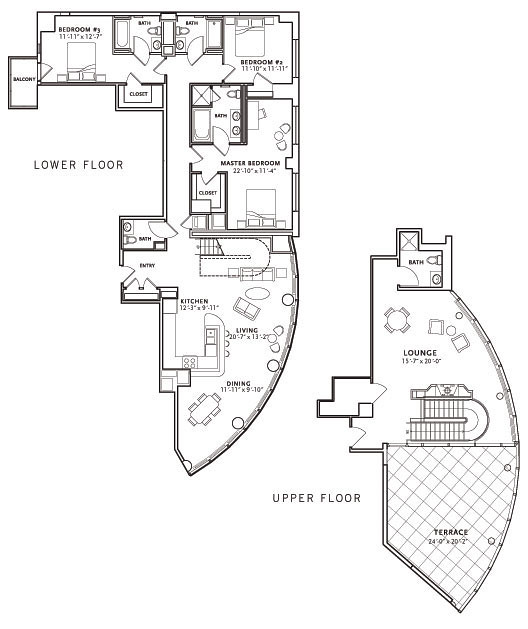This floor plan consists of both a lower and an upper floor. The lower floor, depicted on the left side of the plan, features a balcony, three bedrooms—one of which is a master bedroom—two and a half bathrooms, a kitchen, a living room, a dining room, and a staircase leading to the upper floor. The detailed room dimensions are as follows:

- **First Bedroom:** 11'7" x 11'
- **Second Bedroom:** 11'10" x 11'11"
- **Master Bedroom:** 22'10" x 11'4"
- **Kitchen:** 12'3" x 9'11"
- **Living Room:** 20'7" x 13'2"
- **Dining Room:** 11'11" x 9'10"

The upper floor features a spacious terrace and a large lounge area, supplemented by an additional bathroom. The dimensions for these areas are:

- **Lounge:** 15'7" x 20'
- **Terrace:** 24' x 20'2"

The terrace also appears to have built-in lighting and a surrounding support beam, indicating a well-structured outdoor space. Overall, this is a generously sized and well-appointed home, offering ample living and entertainment spaces across both levels.